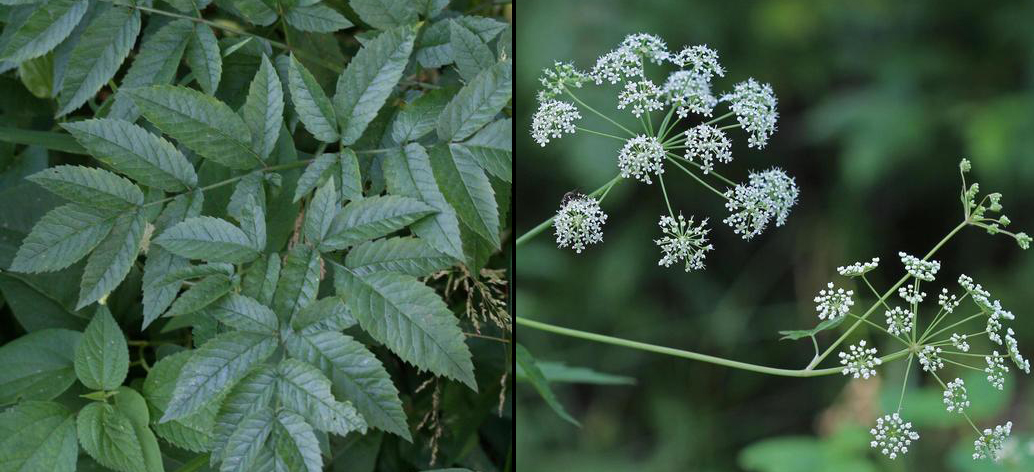This detailed image consists of two close-up photographs of plants, arranged side by side within a rectangular frame. The left-hand side features an up-close shot of a leafy branch, likely poison hemlock. The branch showcases elongated, pointed leaves of a medium green hue, densely packed and overlapping each other. The background is completely focused on these leaves, with a small, indistinct wider plant blurred in the bottom right corner. 

On the right-hand side, the second image portrays the delicate, white flowers of probably Queen Anne's lace, attached to long, thin green stems that branch out into even finer stems. These flowers are very small, each scarcely larger than a dime, forming a lacy, intricate pattern. The foreground is sharp, emphasizing the fragility and fine texture of the flowers, while the background blurs into a mix of green and brown shades, hinting at a forest or shrubbery setting that accentuates the plant's delicate beauty.